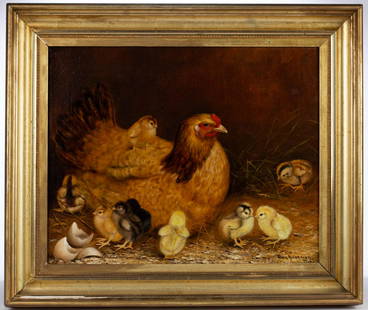The image depicts a richly detailed oil painting set within a thick, ornate gold frame. The painting features a central orange chicken with darker black neck feathers and a red spot on its face, looking off to the right with a clear black eye and a prominent beak. Surrounding the mother chicken are five chicks—four are yellow and dispersed around her feet, with one yellow chick perched on her back. A fifth chick, black in color, stands to the left along with a light orange chick. The scene is one of new life, as scattered broken eggshells are visible on the light beige, grassy surface below them, hinting that the chicks have just hatched. The composition is set against a darkly shaded background, adding depth, and framed within a solid white outer context to highlight the intricate details of the artwork. The dominant palette includes dark browns, yellows, blacks, and the golden hue of the luxuriant frame, creating a visually compelling and warm scene of a mother hen with her chicks.